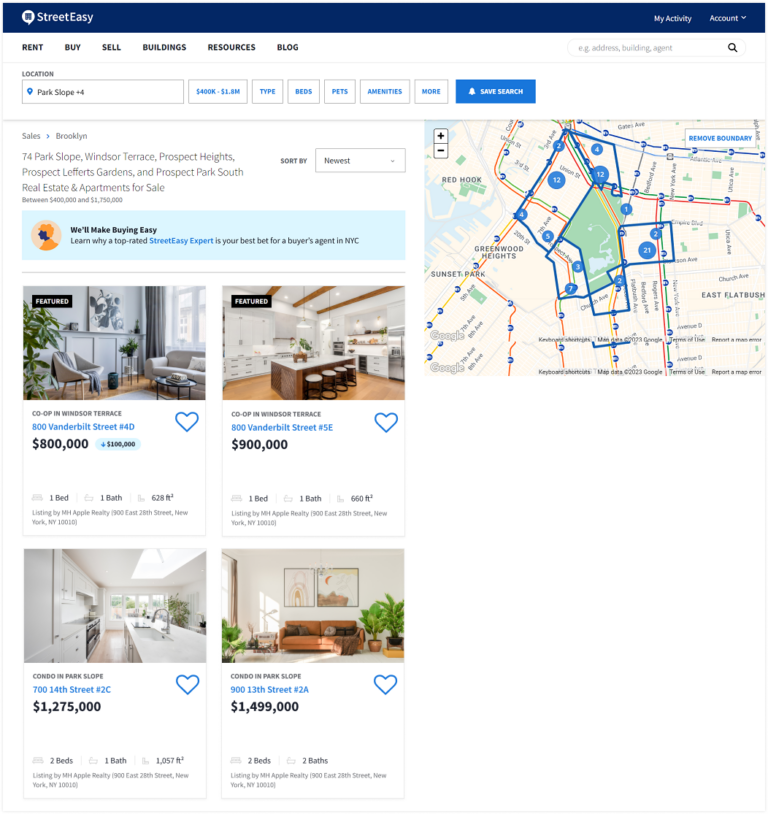On the StreetEasy website, known for facilitating real estate transactions including rentals and sales, the user navigates to the sales section, where they are presented with listings for Brooklyn. Four properties are prominently displayed: two Co-op units in Windsor Terrace priced at $800,000 and $900,000 respectively, both featuring professionally taken photographs; and two Condos in Park Slope, priced at $1.2 million and $1.5 million. The more expensive condo includes two bedrooms and two bathrooms, highlighting the limited yet desirable space available in New York City real estate.